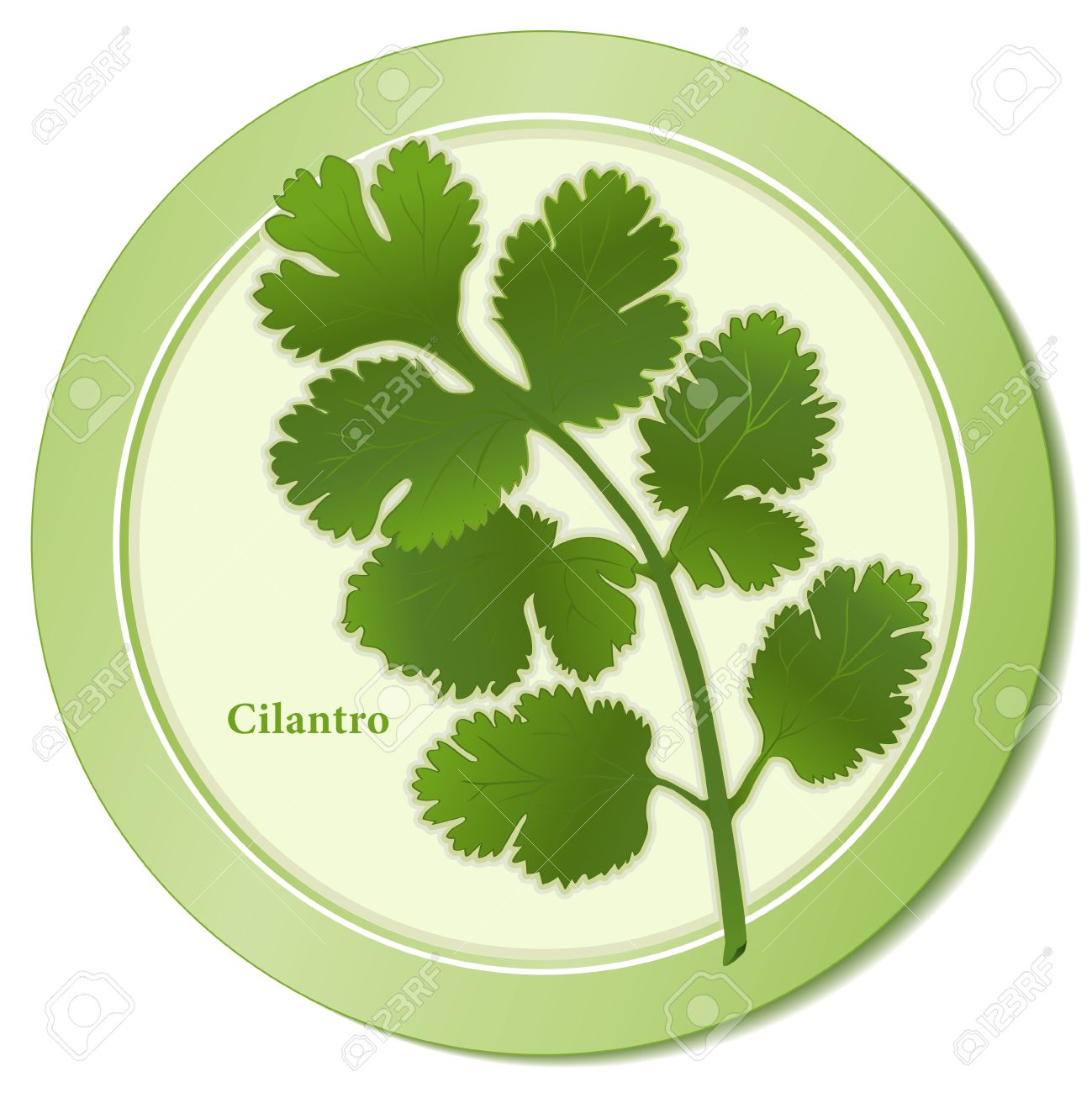The image depicts a stock photo featuring a circular plate with a distinct two-tone design. The outer rim of the plate is a vivid green, while the inner section is a light lime yellow or beige. Positioned in the center is a detailed green cilantro leaf, curving from the bottom right to the upper left. This leaf features seven distinct leaflets on its branching stem. To the left of the cilantro leaf, slightly towards the bottom of the plate, the word "cilantro" is written in thin, green text. Surrounding the plate, the white background includes watermark overlays consisting of the alphanumeric code "1, 2, 3, RF" and a small camera icon, indicating this is a sample stock image.